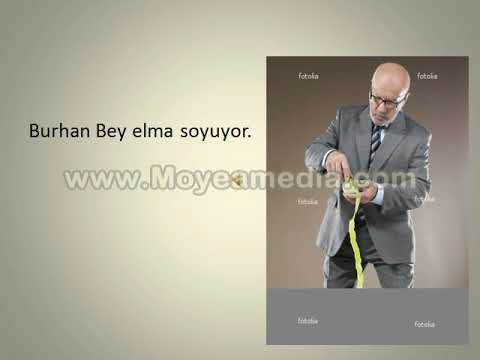This image appears to be an exercise from a language learning book. The top half features a beige or metallic brown background with the bold black number "4" followed by the text "Hangi Resim Arıyor, Telefon Ediyor?" which translates to "Which picture is calling, on the phone?" in English. The phrase ends with a question mark. Below this text, there are three separate pictures each labeled with a letter: A, B, and C. 

- Picture A shows British money.
- Picture B features a young child dressed in pink, holding a cell phone to their ear with a pacifier in the mouth.
- Picture C depicts someone cutting into a red onion.

The three pictures are arranged in a row across the bottom of the image, indicating a multiple-choice format. The image contains various colors including off-white, black, yellow, orange, tan, pink, blue, maroon, and white, suggesting it is designed to be visually appealing and informative. The overall style of the image resembles a PowerPoint slide, contributing to its educational context. The image also contains web text: "www.moyamedia.com," possibly indicating the content’s source.